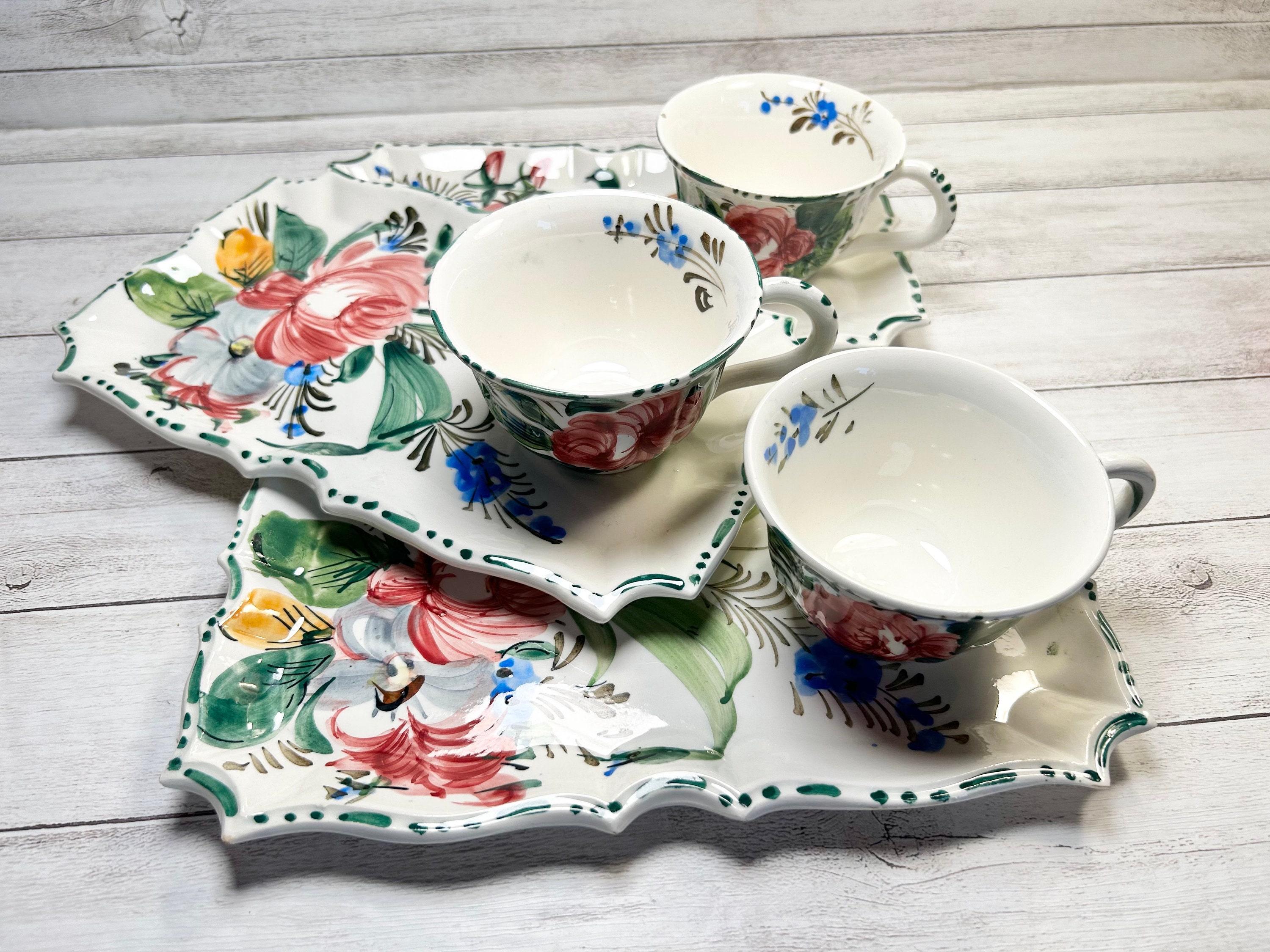The image depicts three white, rectangular plates with extensive and colorful floral designs, including pink and blue flowers and green leaves. These plates, each featuring a matching teacup, are arranged on a wooden table with horizontal slats. One plate is stacked atop the other two at an angle. The teacups mirror the plates' floral motif, with vibrant flowers adorning the exterior and a sprig of blue flowers detailed on the inside. The cups have wide rims, contributing to an overall look that is both antique and elegant. The composition highlights the intricate patterns and harmonious design of the dishware set.